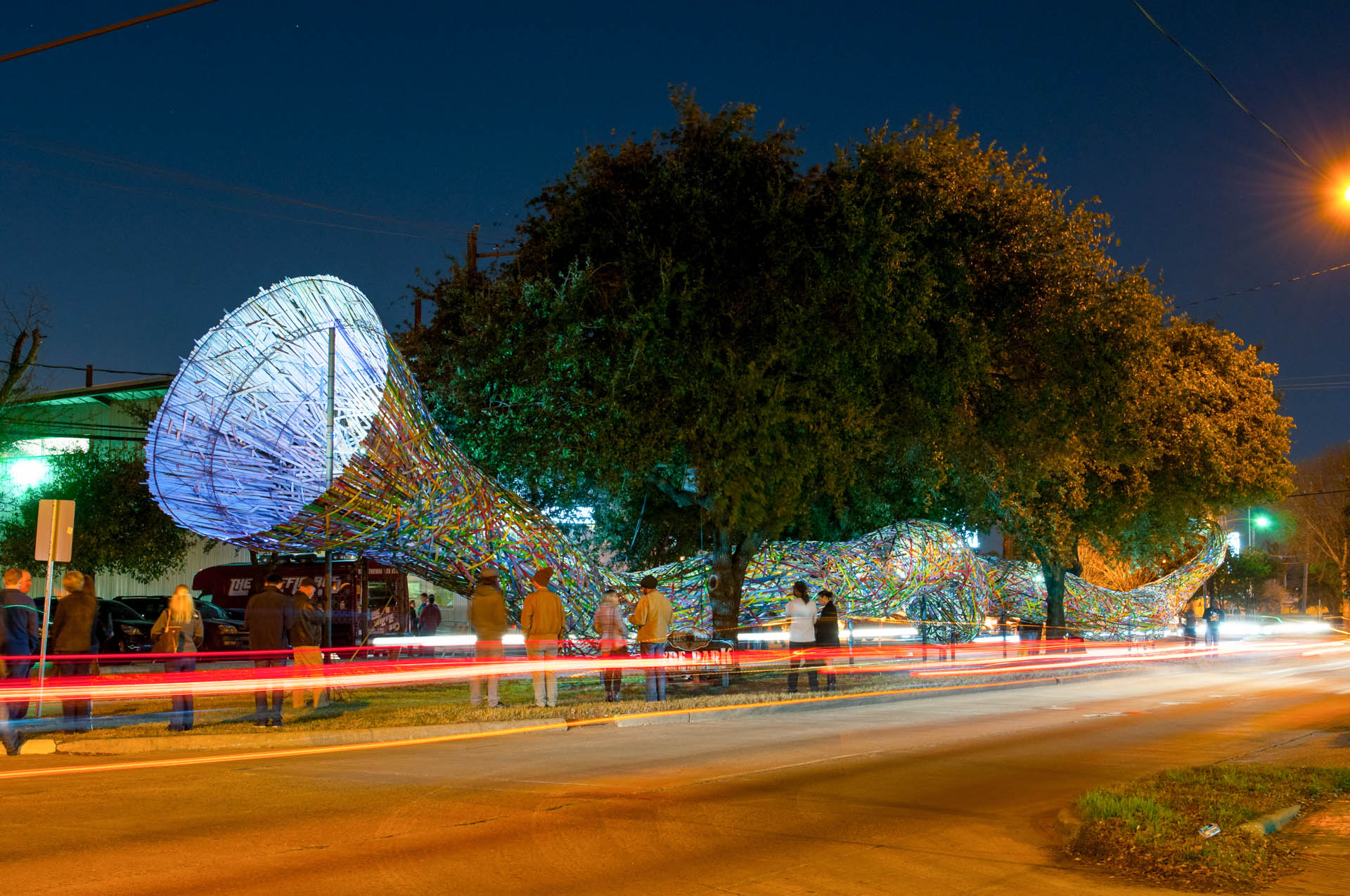The image captures a vibrant and dynamic open-air modern art exhibition set in the middle of a two-laned, tree-lined street at night. Dominating the scene is a large, intricately designed sculpture that resembles a multi-colored, tubular figure with an impressive open circular mouth, reminiscent of a musical instrument like a trumpet. This artistic installation is crafted from an array of vividly colored lines and wires in yellows, blues, greens, and reds, creating a striking, hollow, and wavy structure that spans the entire block. The sculpture stands under several large trees with abundant green leaves, adding a natural canopy to the urban setting. Surrounding this eye-catching piece are numerous onlookers, indicating the artwork has drawn a significant crowd. The street itself is devoid of moving traffic, although some cars are parked on the far side. The atmosphere is illuminated by ambient streetlights, and there are glimpses of red and yellow lights, possibly from passing cars or intentional lighting effects for the exhibit. In the background, a small building is visible, and overhead, electrical wires cross the scene. A green traffic light glows in the distance, adding to the urban nighttime ambiance.